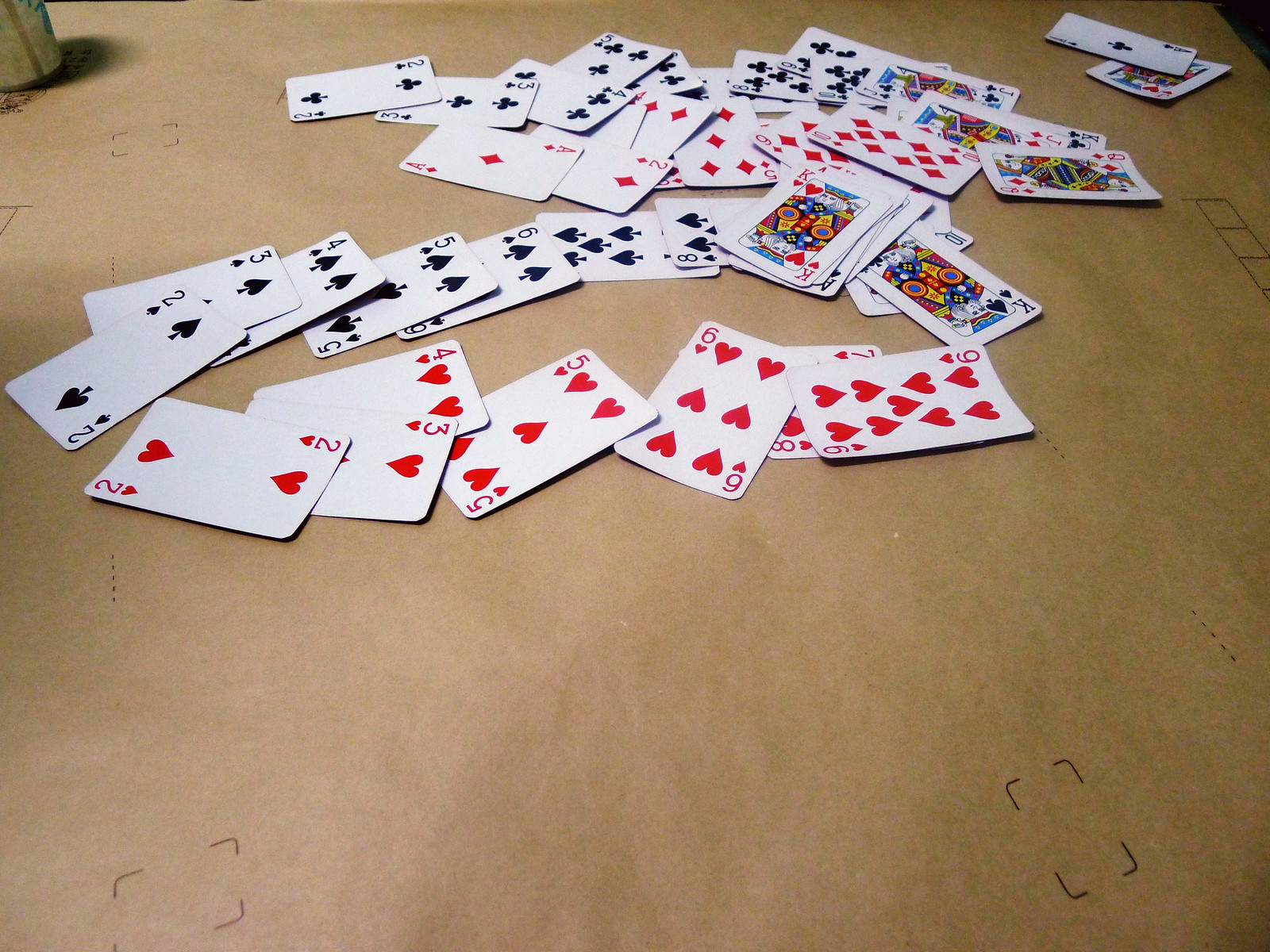This photograph features a brown paper tabletop scattered with numerous black lines. At the bottom of the image, a neatly arranged sequence of playing cards is displayed in two rows. The first row showcases the hearts suit sequentially from the Two of Hearts to the Nine of Hearts, arranging as Two, Three, Four, Five, Six, Seven, Nine, and Eight of Hearts. Parallel above this row is another lineup featuring the spades suit, progressing as Two, Three, Four, Five, Six, Seven, and Eight of Spades.

A pile of cards is placed above these two rows, prominently featuring a Queen of Hearts and a King of Spades on the top of the clutter. There is a mix of cards from different suits within this pile, including Two, Three, Four, and Five of Clubs; Ace, Two, Four, Five, Nine, and Ten of Diamonds; Queen of Hearts; Eight and Nine of Clubs appearing twice; and a Jack of Clubs.

In the top right corner of the image, two cards are set apart from the rest: the Ace of Clubs and the Jack of Hearts. The right side of the paper shows three hand-drawn squares, adding to the casual, cluttered aesthetic of the scene.